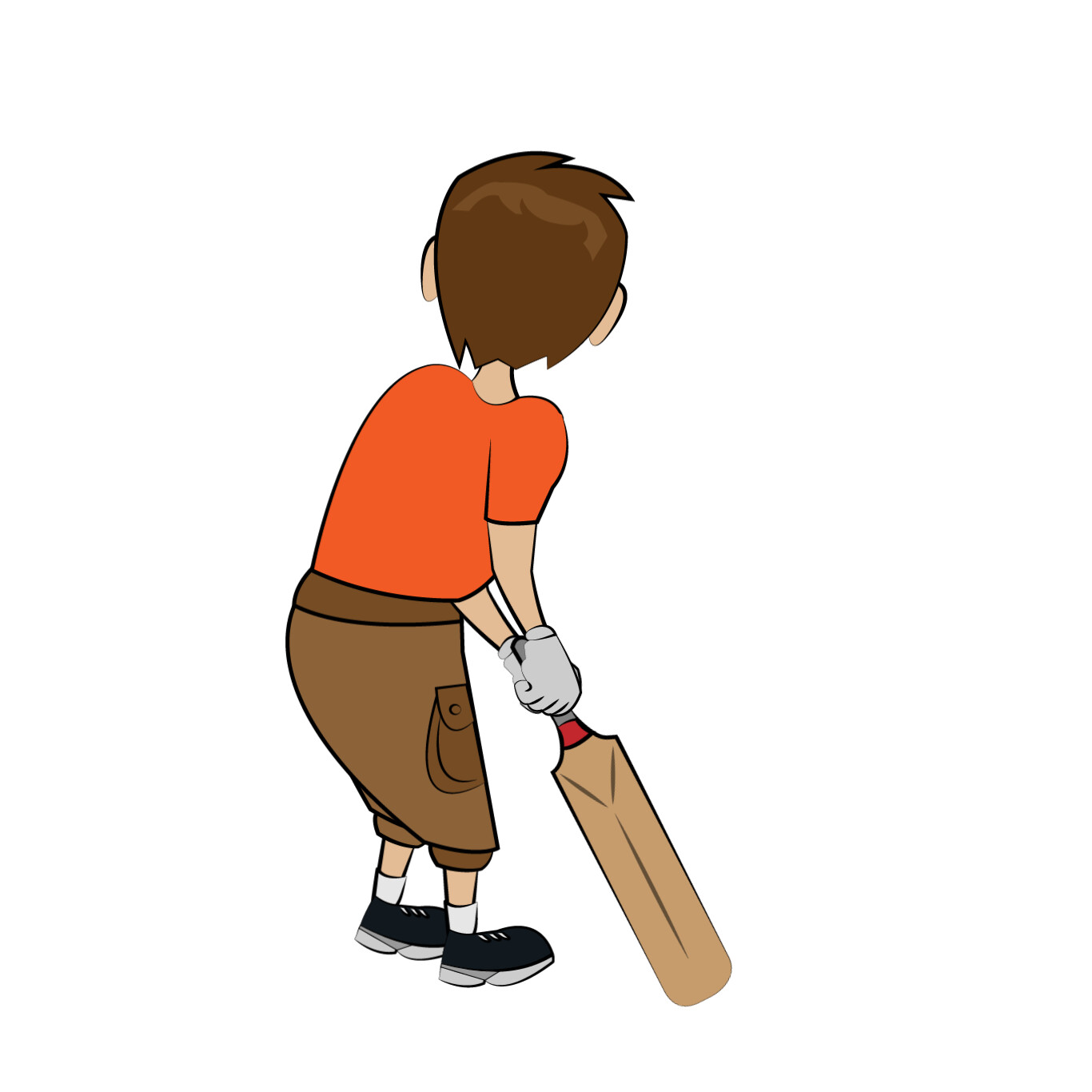This computer-generated illustration, rendered in a simplistic comic book style, captures the rear view of a young boy standing against a featureless, solid white background. The boy has shaggy, medium-length brown hair with two distinct tufts at the top, and flesh-colored pink ears visible from the back. He is dressed in an orange short-sleeved t-shirt and brown cargo shorts that fall just below his knees, featuring a pocket with a snap on the side. His feet are clad in black sneakers with white soles and socks. Notably, he wears white gloves and holds a small cricket bat with a red and gray handle, the wooden bat pointing downwards. His body is positioned with his right shoulder slightly angled to the right side of the image, his arms hanging straight down in front of him as he stands facing away from the viewer.